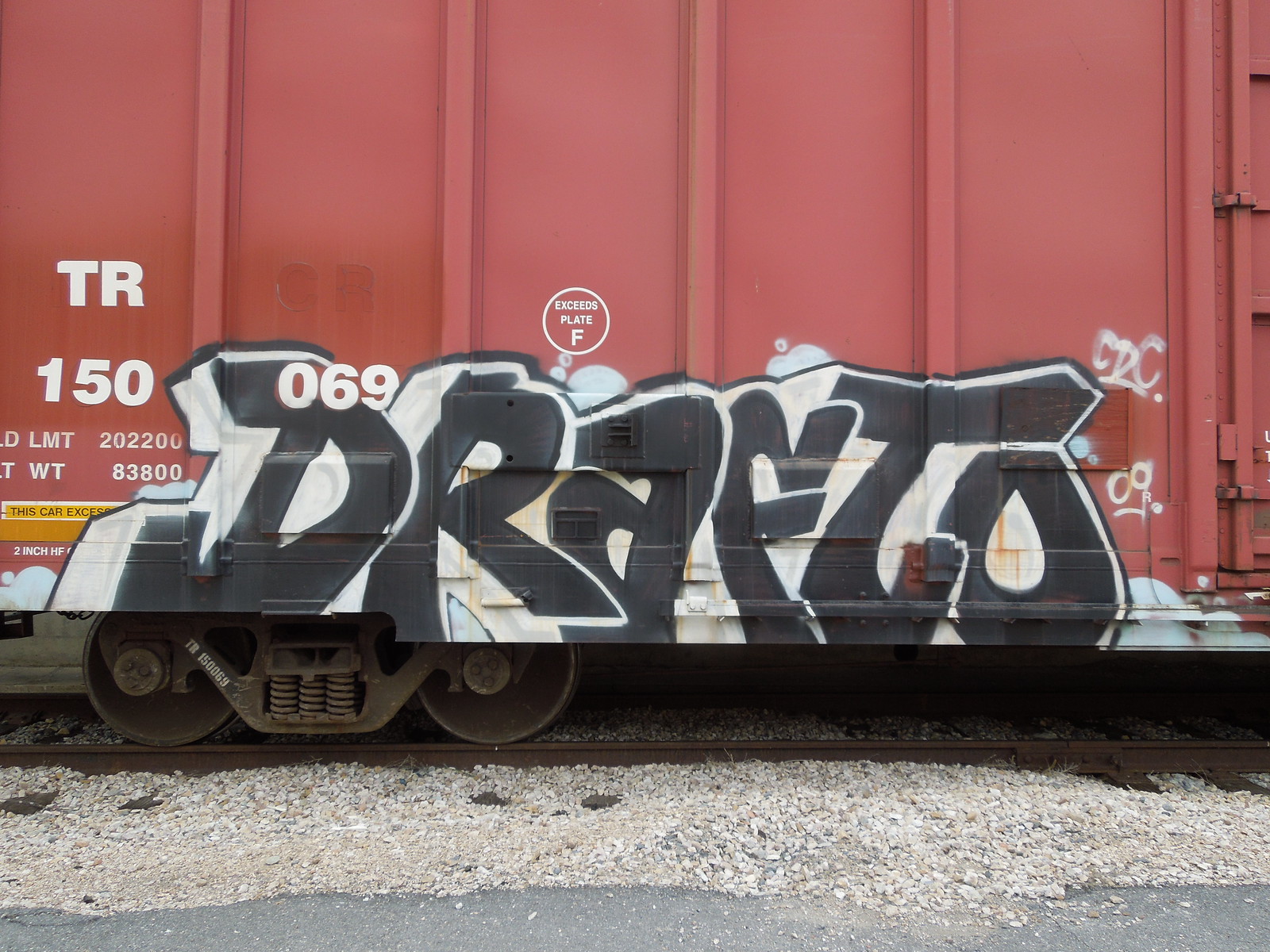This image captures a close-up view of a light red train boxcar adorned with various graffiti and markings. On the far left corner of the car, the white text reads "TR-150", all against the backdrop of the car's vertical slats. Dominating the lower third of the side panel is a large graffiti tag in bold black letters outlined in white, spelling out "DRAFTS", with the letters "A" and "F" in lowercase and the rest in uppercase, giving it a dynamic and artistic appearance. To the right of this prominent tag, there are smaller white graffiti tags displaying "CDC" and "09". Below the train car, the ground is covered in light-colored gravel, along with a visible strip of asphalt and the grey, slightly rusted wheels of the car.